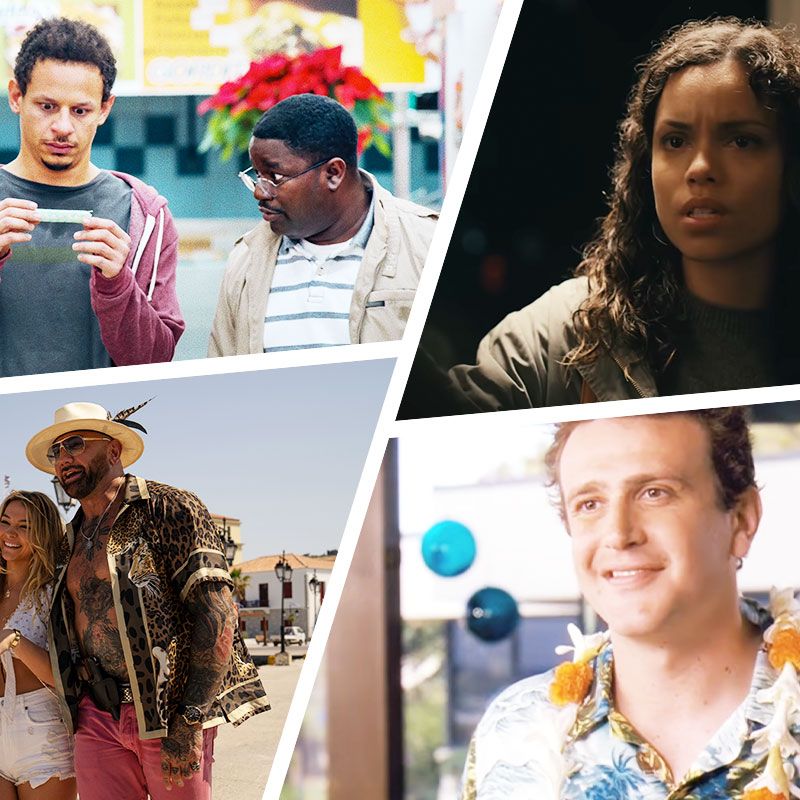This collage consists of four distinct but interconnected photographs arranged in an unconventional, geometric manner with white lines between them. In the upper left, two young men, one black and one white, stand closely together. The white man is holding an object that appears to be a pregnancy test, and both display expressions of curiosity and surprise. The black man, wearing glasses, peers over the rims at the object, and it seems they are in a store or shop setting. Moving to the upper right, a dark, moody photograph shows a Hispanic woman with wavy, shoulder-length hair wearing a coat. She gazes forward with a concerned look, her surroundings indistinct. In the lower left, a lively image depicts a couple basking in a sunny, resort-like atmosphere. The man, heavily tattooed and adorned with a gaudy chain and pendant, wears pink shorts, a leopard-print shirt open at the front, sunglasses, and a feathered hat. The woman beside him, clad in a bikini top and cut-off jean shorts, also smiles brightly. Finally, in the lower right, a white man donning a Hawaiian shirt and a floral lei appears to be on vacation. With sandy brown hair, an earring in his right ear, and a leisurely smile, he looks off into the distance, indoors with a blurred background.